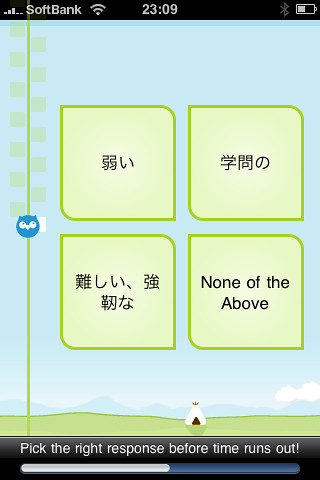The image is a detailed screenshot of a smartphone displaying a language game. The phone's interface shows standard elements such as a black bar at the top, which includes cell service bars, the carrier name "SoftBank," the time "23:09," a half-full battery indicator, and a Bluetooth icon. The bottom of the screen also features a black bar.

The main content of the screen has a light blue background resembling the sky, with a green vertical line on the left side. There is a small owl emoji positioned centrally. Below this, towards the bottom of the screen, the phrase "Pick the right response before time runs out" is displayed above a blue and white progress bar indicating the time limit for the game.

The game interface contains multiple white-bordered green squares arranged in the middle of the screen. Each square contains text in some form of Asian script, with one option clearly labeled in English as "none of the above." Additionally, the bottom part of the background showcases a ground motif with a tiny teepee and patches of green grass against the blue sky with scattered white clouds. This setup indicates that the user needs to select an option by tapping one of these squares before the timer runs out.